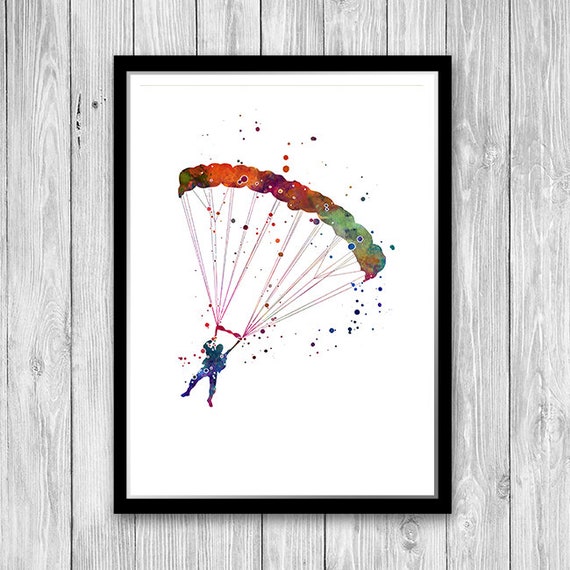This image captures a small painting on a white wooden wall, where the grain of the wood subtly shows through the thin layer of paint. Encased in a simple black frame with about an inch-wide border, the central focus is a parachutist descending through the sky. The parachutist's body is outlined in blue, with one red foot and one blue foot, and he is falling at an angle toward the lower left part of the painting. The parachute he is using is depicted with numerous colorful sections, including green, orange, and purple, held together by long strings. The background features a white canvas accented with splatters of various colors, adding a dynamic and vibrant element to the scene. The overall style suggests a watercolor approach, enhancing the painting's fluid and lively atmosphere.